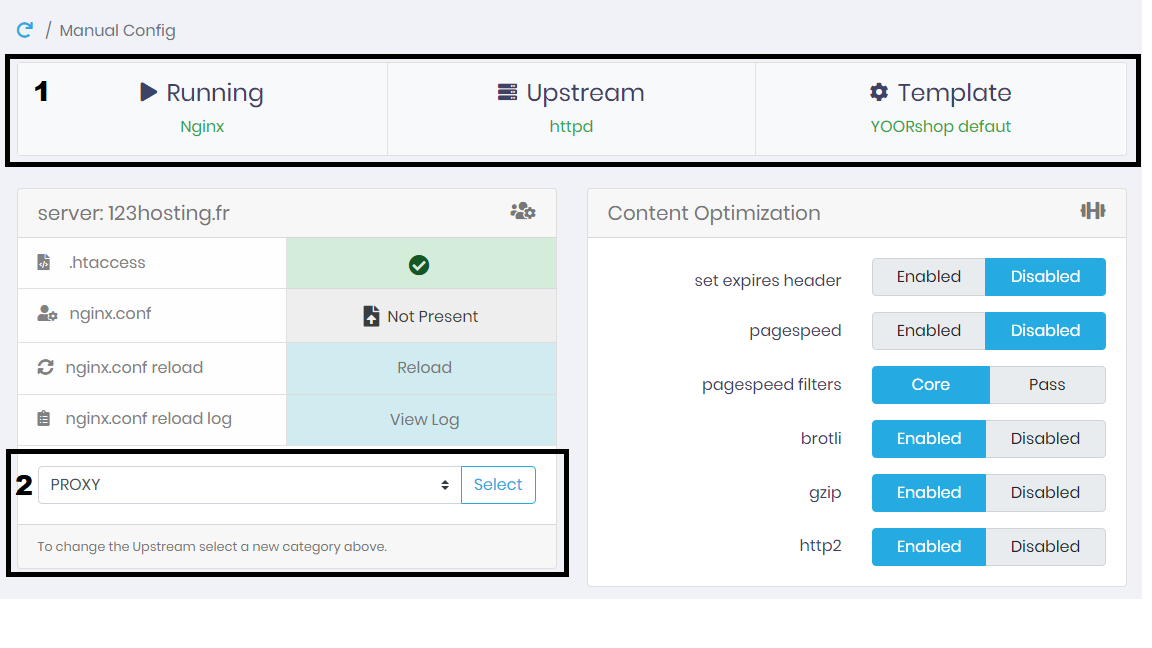Screenshot of a web interface: In the upper left-hand corner, a refresh icon is visible next to the text "#manual config." Across the top of the screen, a horizontal box is segmented into three tabs labeled "Running," "Upstream," and "Template." Below this main section, there are two distinct boxes. The first box is labeled "server123hosting.fr," while the second is titled "Content Optimization." Under a search tab named "Proxy," there's a notation "2." 

Within the "Content Optimization" section, there are six toggles, each allowing the user to enable or disable specific optimizations. When toggled on, the switches turn blue.